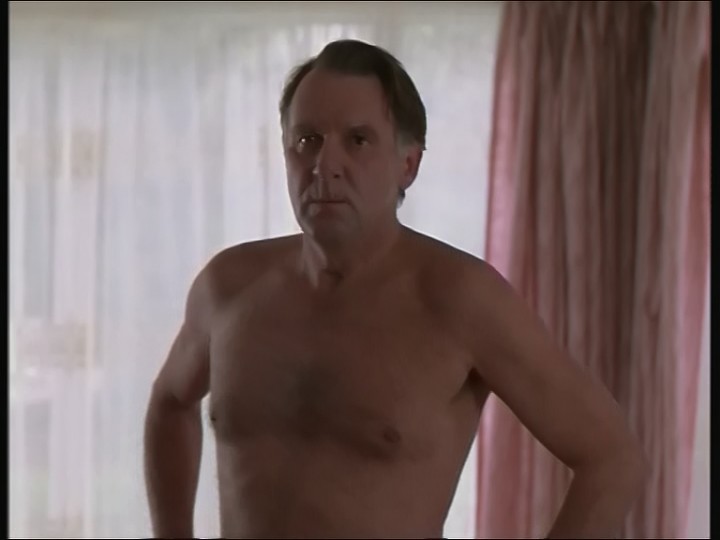This photograph depicts the upper half of a shirtless older man, identified as the actor Tom Wilkinson. His hair is short, predominantly dark brown with hints of gray around the ear level. He is situated slightly in shadow, imparting a serious and earnest expression as he gazes slightly to the left of the camera. His posture suggests that his arms are positioned on his hips, though they're not fully visible to confirm this. The background features a contrast of curtains: white, sheer ones to the left, and pinkish-salmon ones tightly bunched on the right, with a glimpse of outside light and trees filtering through the translucent fabric. The lighting in the room seems to be ambient and natural, lending a soft, dim illumination to the scene without pronounced shadows or glares. Thin black horizontal and vertical lines frame the image.